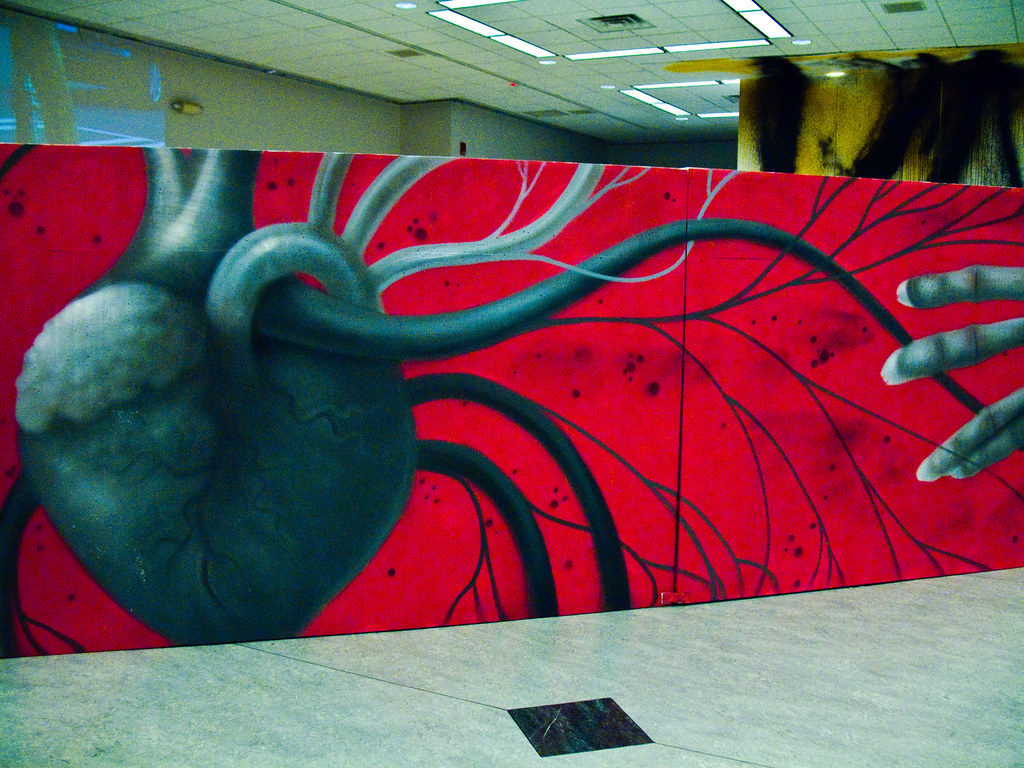The image depicts an indoor photograph of a room featuring a prominent, large-scale mural with a vivid red background. The mural spans a significant portion of the wall, which does not reach the ceiling. Dominating the left side of the mural is a strikingly detailed gray and black human heart, large enough to cover much of the red background. This heart is intricately painted with prominent black and gray veins and arteries branching out across the red surface. The red background itself is accentuated with grungy, splattered black splotches, adding a dynamic texture that might resemble blood. A significant feature is a painted hand on the right side of the mural, reaching towards the heart. This hand appears to be African-American, characterized by long fingernails and dark-skinned fingers, suggesting a feminine touch.

Above the mural is a ceiling composed of square tiles, interspersed with recessed fluorescent lighting and air-conditioning vents. The ceiling meets a gray wall in the top left corner of the photograph. Below the mural is a white marble tiled floor, grounding the vivid image with its smooth, reflective surface.

In the center foreground of the photograph, there is a black square on the ground, and on the right side of the mural, besides the hand, there appears to be a faint impression of another painting, possibly yellow and black, further extending the artistic ambiance of the space, which resembles a museum or gallery setting.